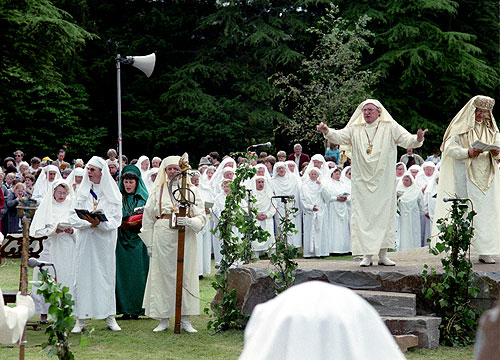The image depicts a Christian religious procession taking place outdoors amidst lush green trees and grass. At the center, there is a prominent stone stage where two priests are standing. The primary priest, wearing a yellow-tinted robe and headscarf, adorned with a large gold chain and medallion, has his arms extended wide. Beside him, the other priest, similarly attired, appears to be reading from a paper. Surrounding them are numerous onlookers, most of whom are dressed in white robes with white headpieces. In the foreground, there is a notable figure in a white robe holding a large wooden staff. Additionally, a woman dressed uniquely in a green robe and headscarf stands out among the crowd. The presence of a very tall light shining on the group adds to the solemnity of the scene. The gathering is marked by an atmosphere of communal singing or speaking, with several white-robed individuals holding books.